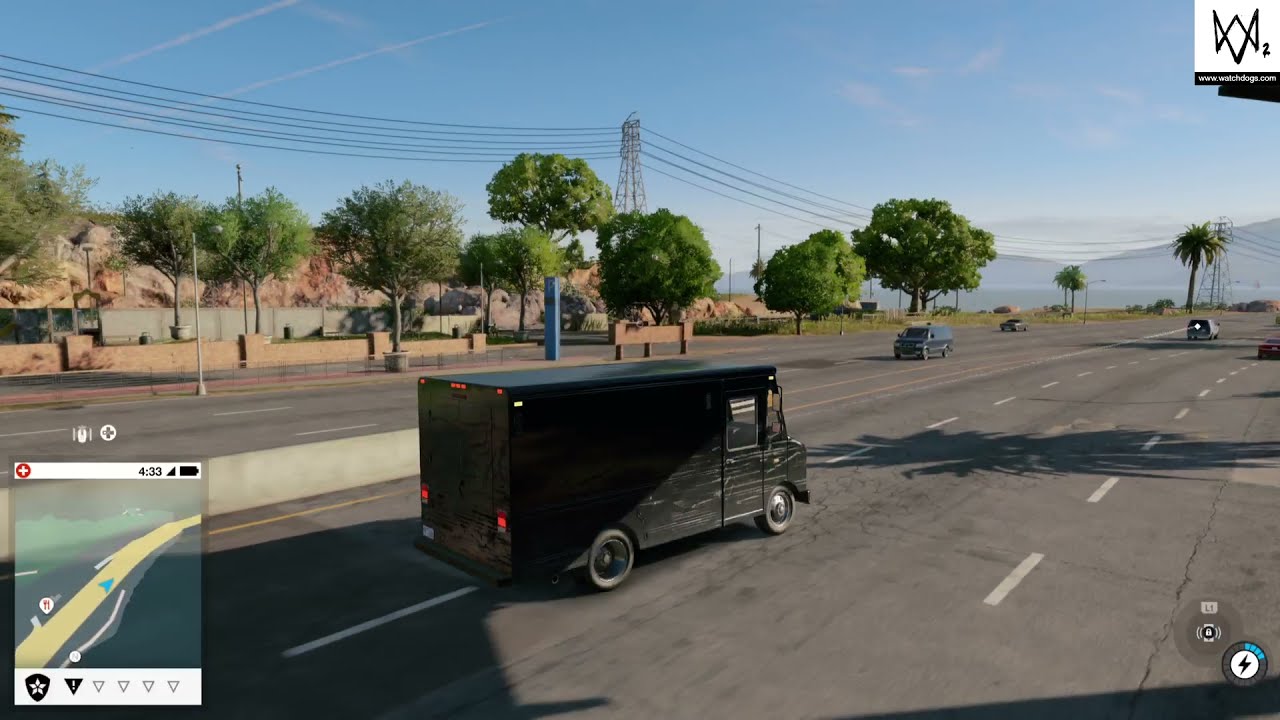In this photorealistic video game screenshot, a large, dark brown or very dark gray delivery box truck, somewhat resembling a UPS or U-Haul truck but without any logos, is traveling down a sunny highway, positioned diagonally across two lanes. The lower left corner of the image features a mini-map indicating the truck's location and route. The highway is lined with trees, including palm trees, and there is oncoming traffic in the distance on the far side of the road. A long tan building is visible beyond the tree line on the left. The skyline showcases a blue sky with light clouds and contrails from jets, with mountains forming the horizon in the background. Electrical power lines stretch from the upper left to the middle right of the image, and a low stone wall, a fence, and a rocky hill appear in the background. Additional game interface elements include a gray circle with a dot, a white circle with a lightning bolt on the lower right, and a white square with a symbol and unreadable white text in the upper right corner.